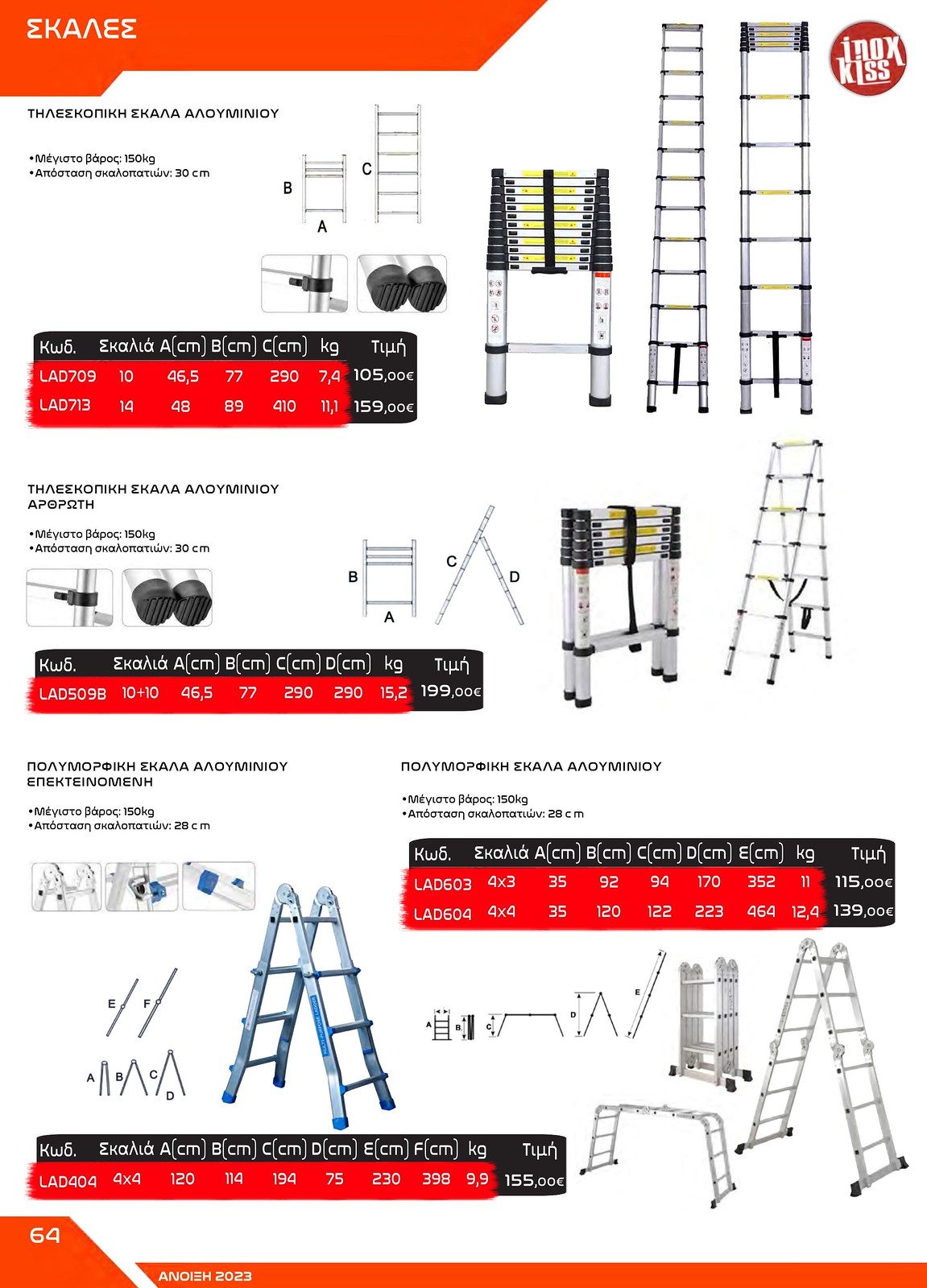This image appears to be an advertisement or instructional diagram for various ladders, demonstrating how they can be assembled and adjusted. The image is not in English and features multiple sections detailing the different attributes and configurations of each ladder. At the top right, an orange banner with white foreign text stretches about two-thirds across the image. Below this banner, there is a compact, wide ladder with silver legs, black upper components, and six yellow steps, along with a depiction of its adjustable height. Lower on the diagram is a similar but shorter ladder with fewer legs. At the bottom left, a silver A-frame ladder with four steps is shown. To its right is an extended ladder with four steps ascending, then six steps horizontally, and another six steps descending, which can also be reconfigured into an eight-step-high A-frame ladder. The diagram also includes red and black graphs and measurements in centimeters and kilograms, suggesting detailed specifications. The ladders are metal, and some have non-slip bases. The comprehensive diagrams and foreign text make it resemble part of an instruction manual, emphasizing the versatility and assembly of various ladder types, including those that can transform into step stools or take multiple shapes.